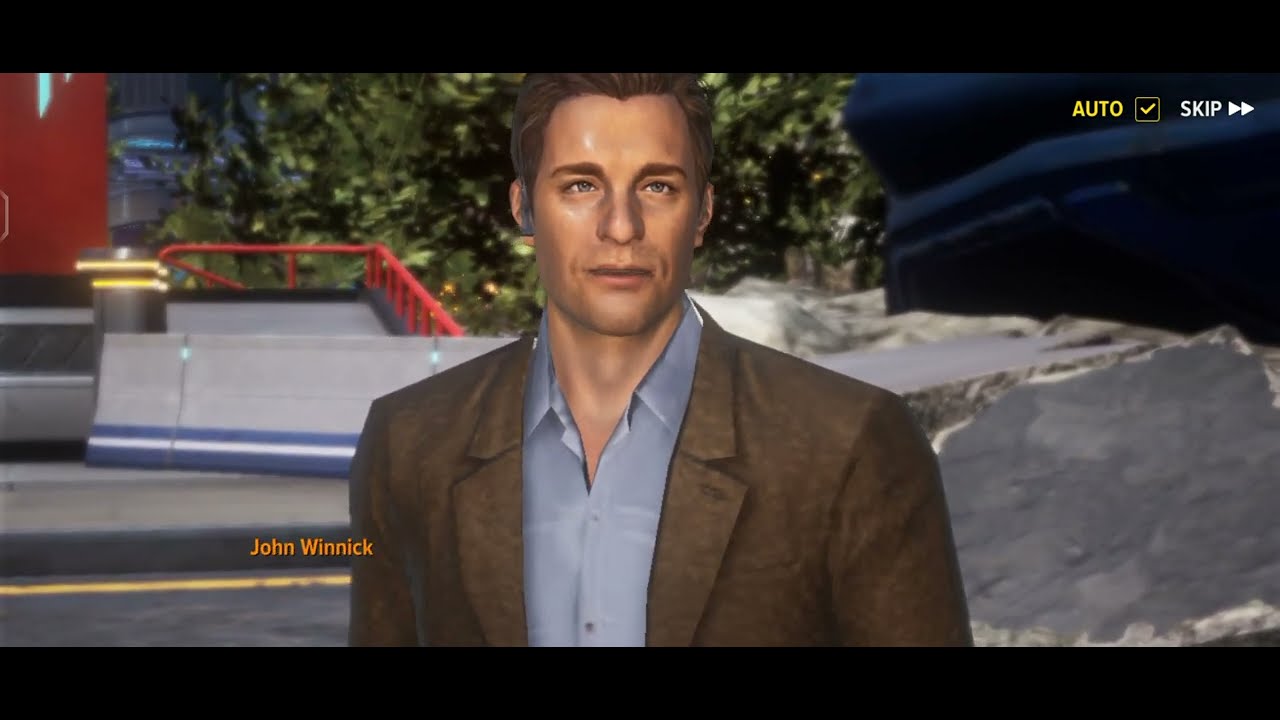This image is a computer-generated screenshot from a video game, featuring a central male character named John Winnick. He appears to be in his late 30s to early 40s, dressed in a professional brown suit jacket and a light blue button-down shirt, with the top button undone. He has slicked-back short brown hair, striking blue eyes, and a strong jawline. The character's name, "John Winnick," is displayed in yellow font near his right shoulder on the left-hand side of the image. The scene is framed by a black border on the top and bottom, with interactive options in the top right corner: a yellow "auto" checkbox and a white "skip" button with a fast-forward icon.

John is set against a background that blends futuristic and natural elements. To his left, there's an entrance to a building with a red railing and a red structure behind it. The ground appears to be concrete with a step visible, and there are green deciduous trees and shrubs nearby. On the right side of the scene, partially obscured, there is a blue structure, possibly part of a building, and some large silver rocks, possibly forming a rock pathway. The entire scene suggests a mix of urban and natural settings, characteristic of the game's aesthetic.